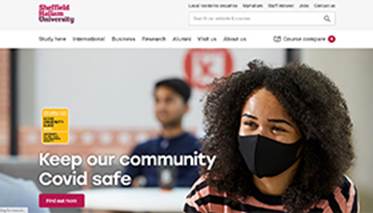On the banner of a web page, the word "Sheffield" is visible next to a search box with a magnifying glass icon. The web page features seven navigation tabs. Below the banner is an image set in what appears to be an office environment. In the foreground of the image, a young woman, who seems to be biracial, is wearing a mask that covers her nose and mouth. She has brown, curly hair and is dressed in a striped shirt featuring peach or pink and black stripes. The text in the image reads, "Keep our community COVID safe." Behind her, a young man stands with his arms crossed, seemingly looking in her direction. There is also a red button beneath the text.